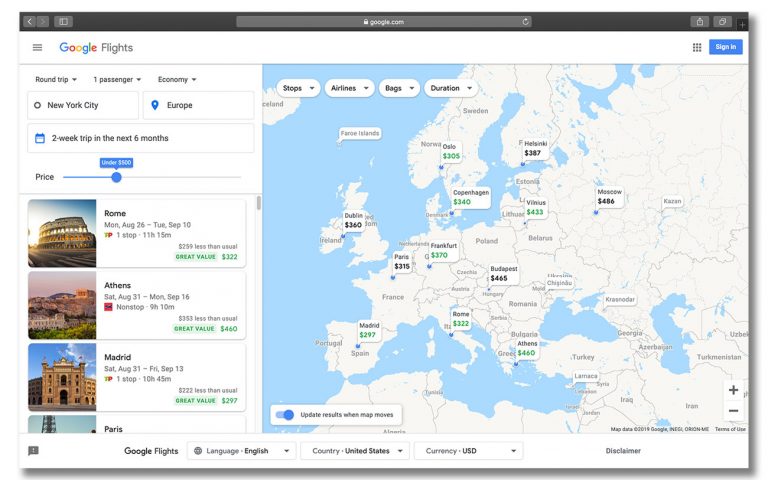Displayed on the web page is an interactive map showcasing various destinations. Positioned on the right side of the screen, the map is detailed with white and blue tones, featuring black lettering that marks the locations and destinations available for selection. Each destination includes an associated cost, with prices varying depending on the location, clearly indicating a range of higher and lower charges.

Accompanying each location is a pertinent image, offering a visual preview of the destination to provide users with a better understanding and sample of the places they can visit. Further down the page, additional information and reference materials are available for those who need more details or assistance.

The interface also features navigational aids such as arrows and a globe icon, which enhance user interaction. Additionally, disclaimers and exclamation points highlight important notices and points of attention, ensuring users are well-informed as they explore the map.